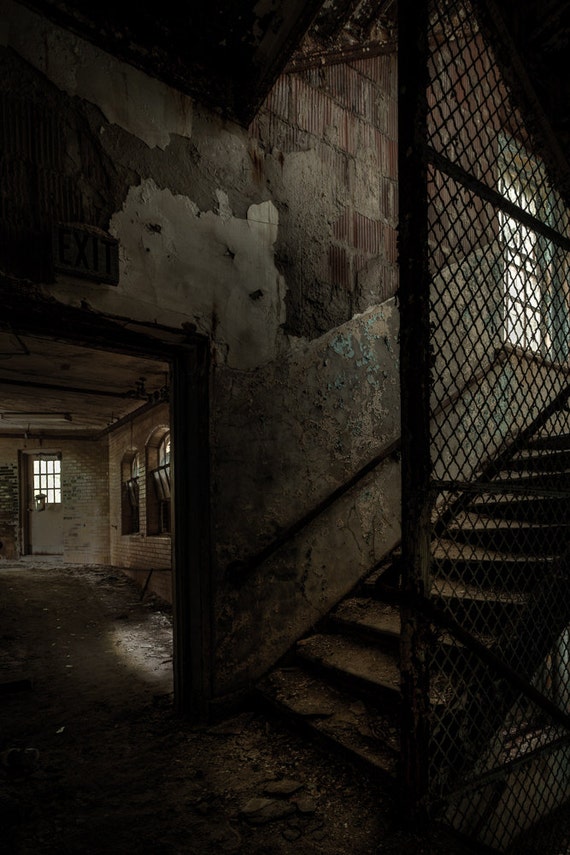The photograph captures a dark and dreary scene of an old, dilapidated building. Central to the image is a filthy metal staircase, cluttered with debris, ascending from the middle of the frame towards the right. Flanking the staircase on its right side is a chain-link fence with diamond-shaped mesh, providing a somber, enclosed feel. To the left, the damaged walls, once painted but now peeling to reveal the underlying block, and a grimy doorway lead to another room. This adjacent room, visible through the doorway, features barred windows—a large one on the right wall and another with a door on the back wall, also secured with bars. The floors throughout are covered in dirt and debris, enhancing the overall sense of neglect and disrepair. The environment is marked by harsh concrete, minimal lighting, and an omnipresent bleakness, suggestive of an abandoned or heavily fortified structure.